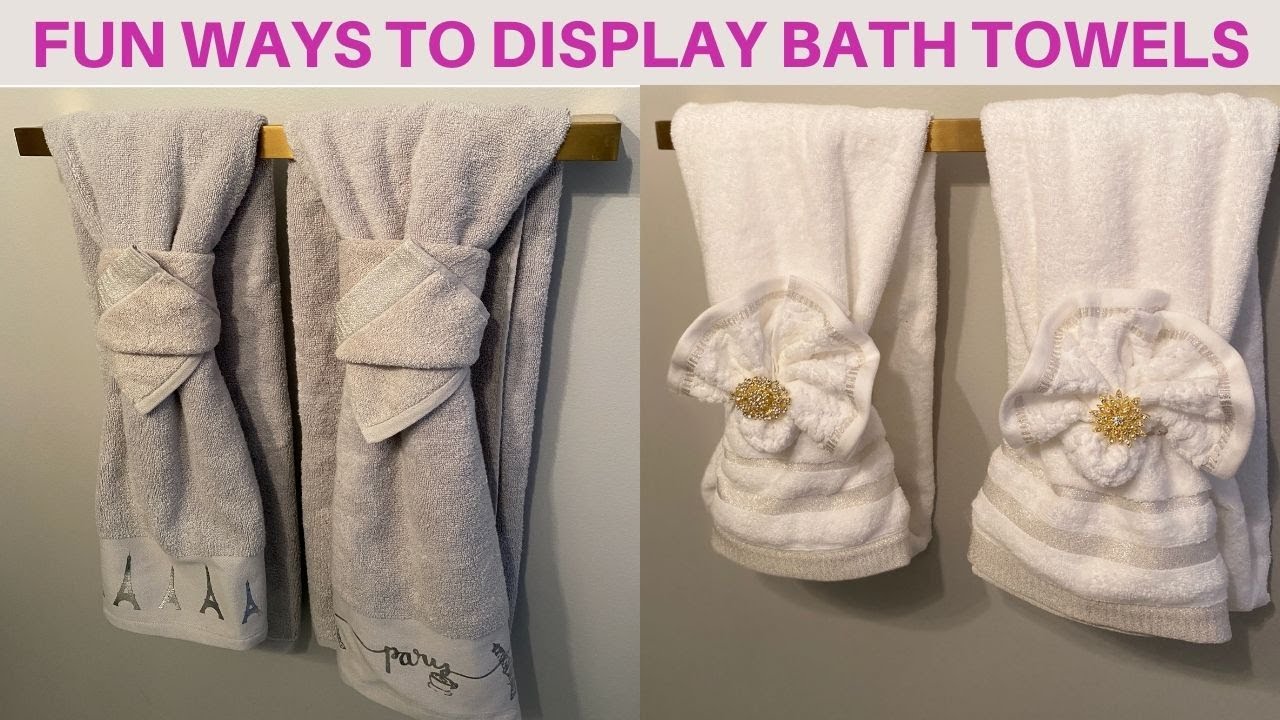The image consists of two side-by-side photograph displays against a brown wall. At the top, a light gray horizontal rectangle features the text "FUN WAYS TO DISPLAY BATH TOWELS" in all caps purple letters. The bottom part showcases two golden bars mounted on the wall, each supporting different towel arrangements. 

On the left, the image displays two light gray towels, artistically tied in the middle by washcloths, forming a unique design that resembles a necktie. The towel on the left features an outline of the Eiffel Tower at the bottom, while the towel on the right is inscribed with the word "Paris". On the right side, the image showcases two white towels with gray trims. These towels are folded so they resemble a flower petal shape, secured at the center by a gold object, possibly a pin. Both towel arrangements demonstrate creative and aesthetically pleasing ways to display bath towels.